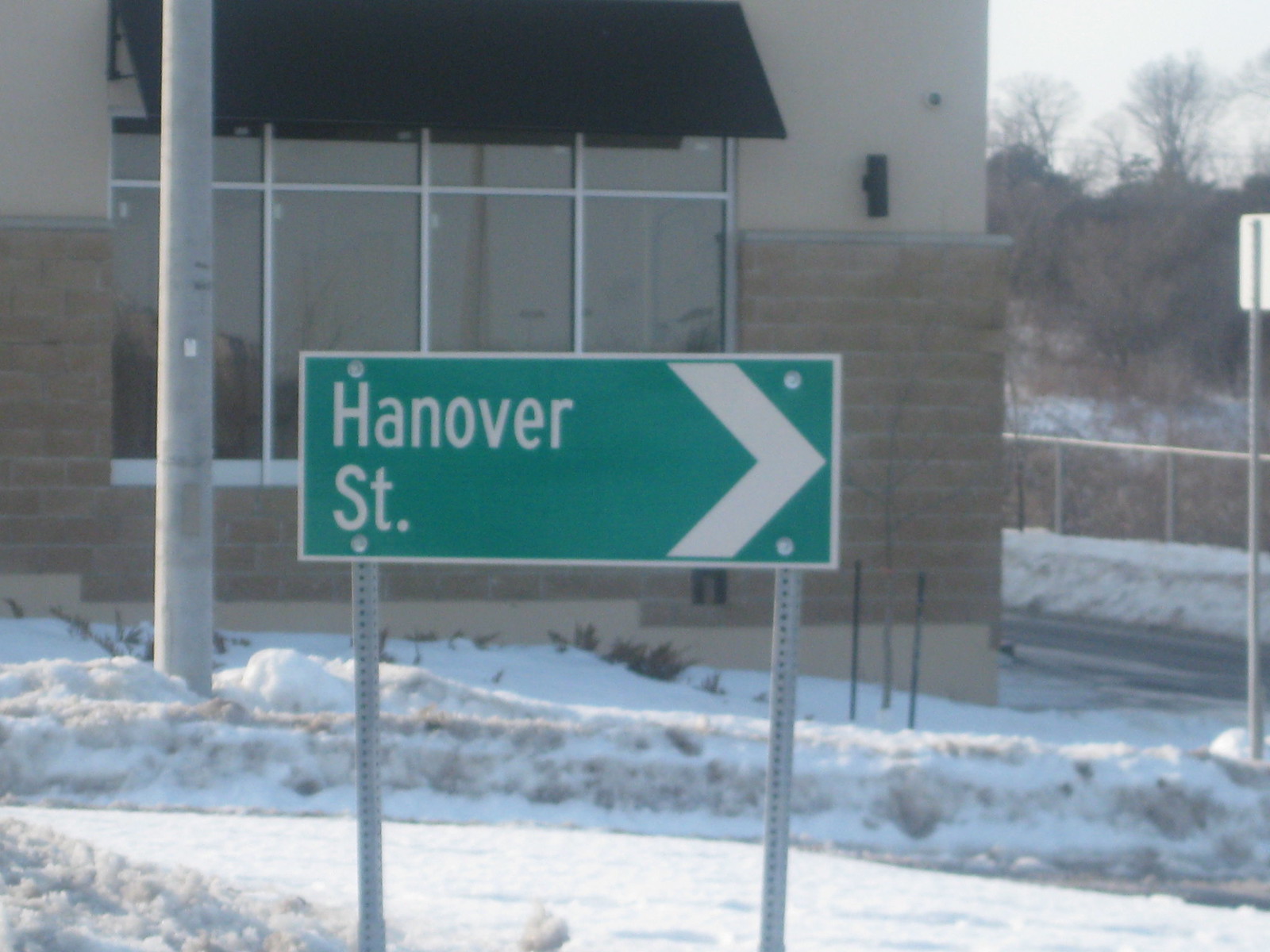The image prominently features a sign with the text "HANOVER" in bold white letters. Below it, there is an abbreviation "ST." written in white, followed by a thick white greater-than symbol on the right side of the sign. The sign itself is outlined with a white border and its corners are precisely 90 degrees.

Behind the sign, there's a stone building. The bottom portion of the building appears to be constructed from darker brown stones, which sit atop a tan-colored concrete foundation. A cement-gray ledge separates the stone base from the tan upper portion of the building. On the right side of the building, there's a cylindrical black light fixture, open at both ends to facilitate illumination.

A window is visible with a unique layout: it is divided into four columns and two rows. The bottom row occupies around 80% of the window's height, while the top row takes up the remaining 20%. Above the window, there is a black awning that is angled to prevent snow and other elements from accumulating on the window.

In front of the building, on the left side of the window, there is a light pole. The ground in the foreground consists of various types of pavement or cement. A fence is present, beyond which there are snow-covered undeveloped lands and woodlands. Snow is visible across the landscape, appearing as if it has been recently moved or disturbed in some areas. The sky is predominantly white, though there are hints of darker shades due to the lighting conditions, suggesting overcast weather.